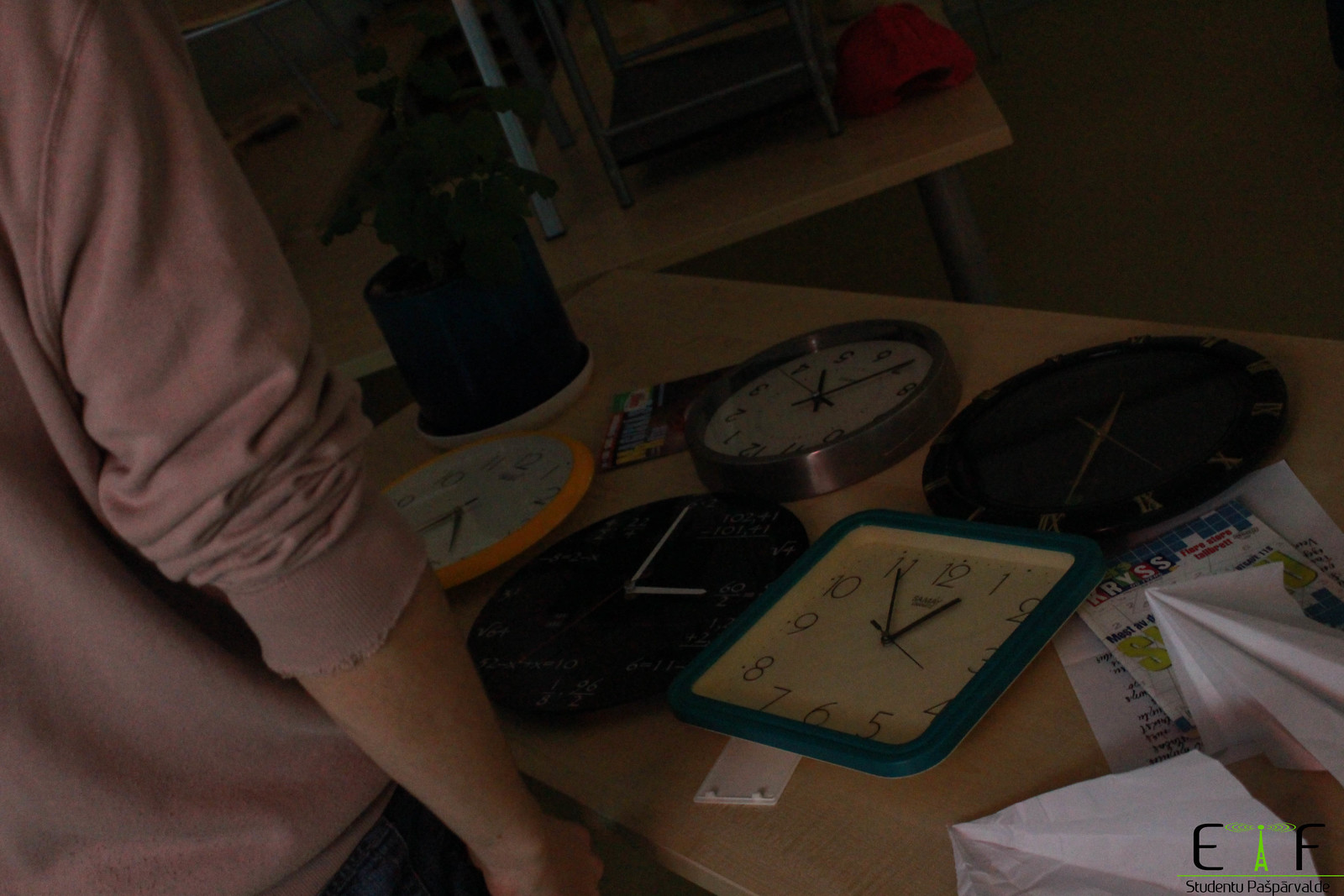In this detailed image, a person in a pinkish long-sleeved sweat top, with sleeves rolled up to the elbows, is intently observing five clocks positioned on a brown wooden table. The individual is partially visible from the back and stands to the left side of the frame. On the table, each clock has distinct features: the leftmost clock boasts an orange rim with a white face, the central clock is entirely black with white hands, and the rightmost clock has a teal blue rim with a yellow face. Additionally, there's a black clock with Roman numerals near the right-hand side and another clock with a brass outline positioned at the top. The table also holds white pieces of paper and what seems to be magazines or documents, as well as a black circular object with a white bottom on the left. Another brown table appears in the foreground, partially in shadow, contributing to the image's depth. The bottom right corner of the image includes the somewhat obscured text “E.A.F. Studento Pasparvalo.”